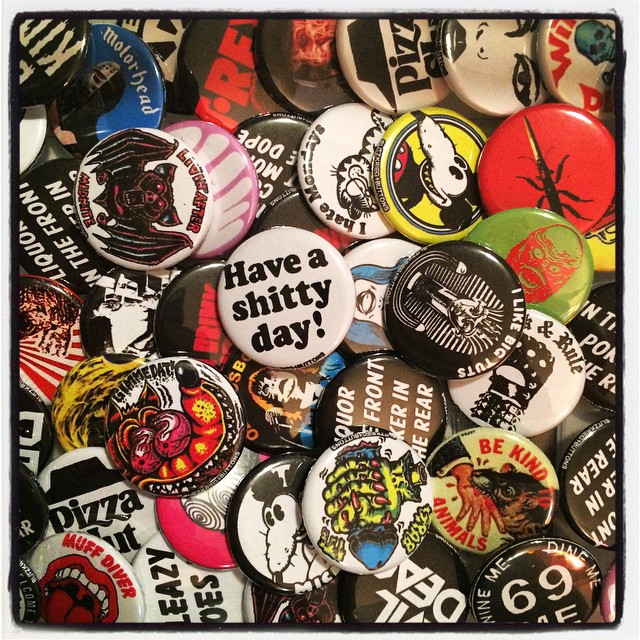The image is a color photograph in a square format, depicting a pile of colorful promotional buttons spread out from edge to edge. These round metal buttons, often worn on shirts or lapels, boast a variety of images and taglines. The scene is framed by a light gray border with a marker-esque black edge. 

At the center of the image is a prominent white button with the black text "have a shitty day." To its right, there's a black button adorned with a white depiction of a pharaoh's burial mask, accompanied by the phrase "I like big tuts." Other noticeable buttons include a red button featuring an insect, a yellow button with an old-style Mickey Mouse, and a button depicting Garfield with the text "I hate Mondays." Multiple Pizza Hut buttons and another that reads "be kind to animals" but shows a rat biting a hand are also visible in the pile. The photograph, capturing the buttons in a realistic, photorepresentational style, highlights their varied, and sometimes irreverent, themes.